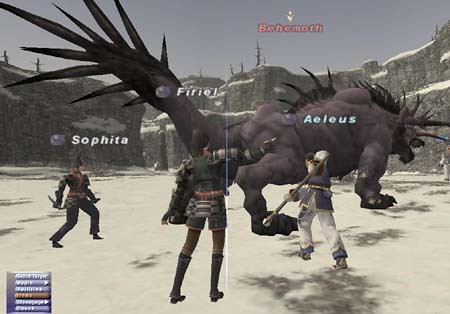In this detailed screenshot from a video game, we see a dramatic scene featuring a large, formidable beast known as Behemoth, facing away from the viewer. The Behemoth is a massive quadruped, brown in color, with an array of menacing spikes along its back, forehead, and tail, which ends in a collection of pointed spikes. It towers over the human figures on the screen, standing at about twice their height.

Centered in the image is a human avatar named Firiel, also facing away from the viewer. Firiel is clad in armor, wearing black boots and has black hair, with shorts and an armored front. She is pointing to the right, adding a dynamic sense of action to the scene. On Firiel's left stands Sofita, easily identifiable by the white text labeling her. Sofita is dressed in a black uniform and wields a dagger in each hand, poised for combat. On Firiel's right is Aelius, also labeled in white text. Aelius is outfitted in white and dark gray armor with white pants and appears to be attacking the Behemoth's leg with his staff.

The background features snow-capped cliffs and a gray sky, lending a cold, foreboding atmosphere to the scene. Further adding to the setting's ambiance is a walled city or coliseum-like structure made of brick or rock, suggesting an arena or battleground where this intense confrontation is taking place. The sandy ground underfoot hints at a desolate and harsh environment, completing the image of this epic and perilous video game moment.